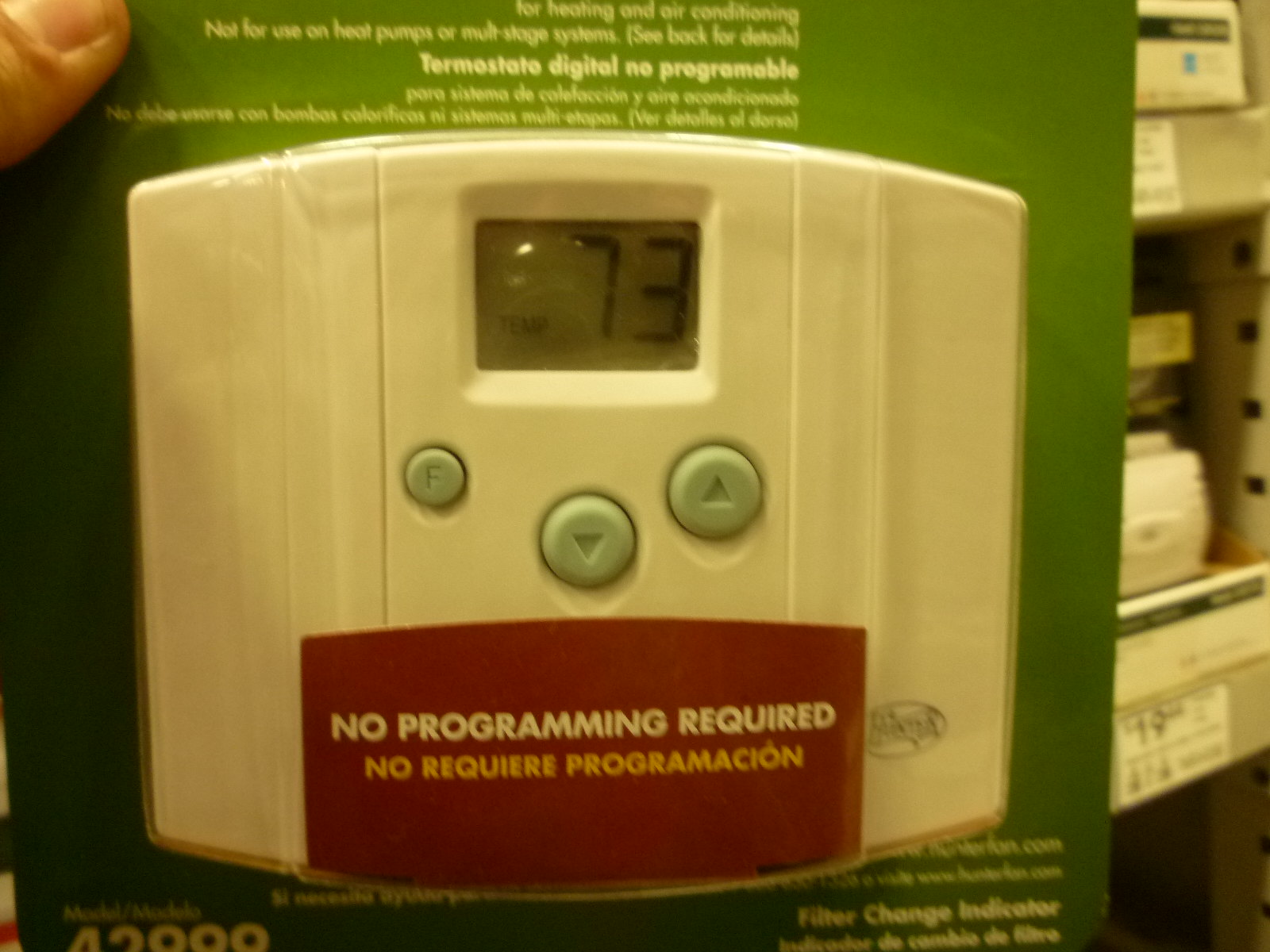The image features a "No Programming Required" digital thermostat designed for heating and air conditioning systems, excluding heat pumps and multi-zone systems. The thermostat is enclosed in a gray cardboard backing with a plastic cover. At the top of the packaging, there is text indicating its usage limitations and instructions to see the back for details. The thermostat is described as "digital" and "non-programmable," with an additional notice in Spanish, though the text is blurry.

The display of the thermostat in the image shows a temperature example of 73 degrees and a time or setting of 10. The thermostat itself is made of white plastic and features light blue buttons, including a small button labeled "F" on the left, and buttons for "Up" and "Down" positioned diagonally. There is a brand logo on the bottom right corner of the thermostat.

The bottom right of the packaging mentions a "filter change indicator," although the bottom left part, which presumably contains additional details or a model number, is cut off. The background reveals store shelves typical of a hardware store, with price tags visible on the lower shelves, one of which shows "$19.44" but is not clearly associated with a particular item.

The thermostat package is being held by someone, with their thumb visible at the top left, showing short nails and cuticles that need some attention. A website is also listed on the box, but it is blurry and unreadable.